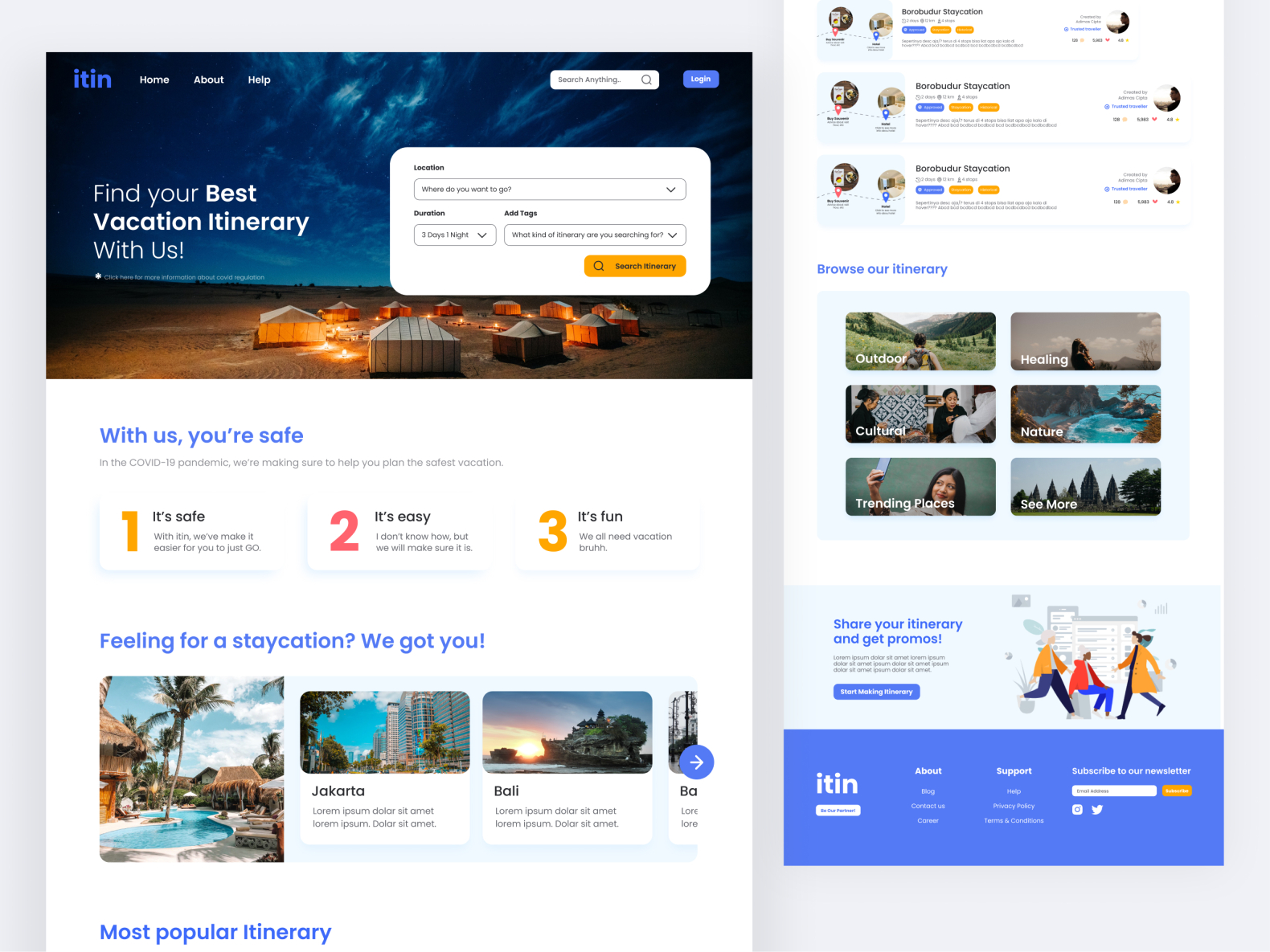The image shows a detailed mock-up of the user interface for a vacation itinerary app named "It's In" (spelled as I-T-I-N). The interface appears to be designed for both tablet or laptop screens and mobile phones.

On the left-hand side, the interface features a prominent top banner with the action text "Find your best vacation itinerary with us." This banner showcases an image of a camping scene set in a desert landscape. Embedded within this banner is a white rectangular input box where users can enter their desired location, duration of stay, and select relevant tags to specify the type of itinerary they are looking for. Accompanying this input box is a "Search" button.

Below this banner, the app emphasizes a commitment to safety during the COVID-19 pandemic, assuring users that planning a vacation with "It's In" is safe, easy, and fun. There are brief explanations provided under each of these assurances.

On the right-hand side, there is a narrower screenshot that appears to be tailored for mobile phone screens. This section highlights various staycation options in Borobudur, an iconic location in South Asia or India. The options include details on who created them. Following this, the text "Browse our itinerary" prompts users to explore further. There are six bubbles, each accompanied by an image representing different categories such as Outdoor, Healing, Cultural, Nature, Trending Places, and a "See More" option.

Lastly, the mock-up hints at additional features accessible by scrolling further down, including a directory for more detailed exploration.